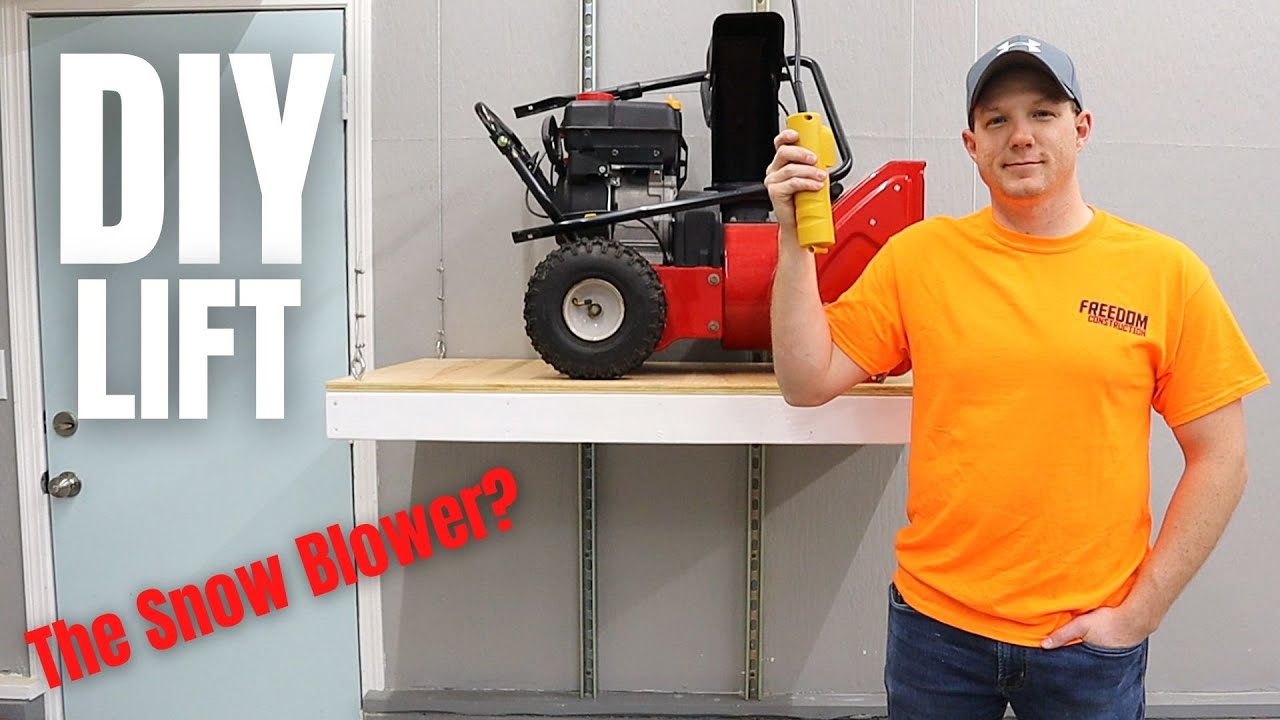The photograph captures a man standing in front of a wooden shelf contraption described as a "DIY lift," with the text "DIY lift" written in white on the left side. Below this, in red text and at an angle, the words "The snowblower?" are visible. The man, who appears to be in his late 30s, is dressed in an orange t-shirt emblazoned with the word "Freedom," blue jeans, and a gray cap. He is holding a yellow object, possibly a handle or a battery that may be connected to the red mechanical snowblower on the lift. The snowblower has a small engine and what seems to be two wheels. The setting features a gray cinderblock wall behind the man and the lift. Wires can be seen trailing down from the lift, indicating complexity in its design. The rightward portion of the photograph is dominated by the large, red snowblower, adding to the overall industrial and mechanical aesthetic of the scene.